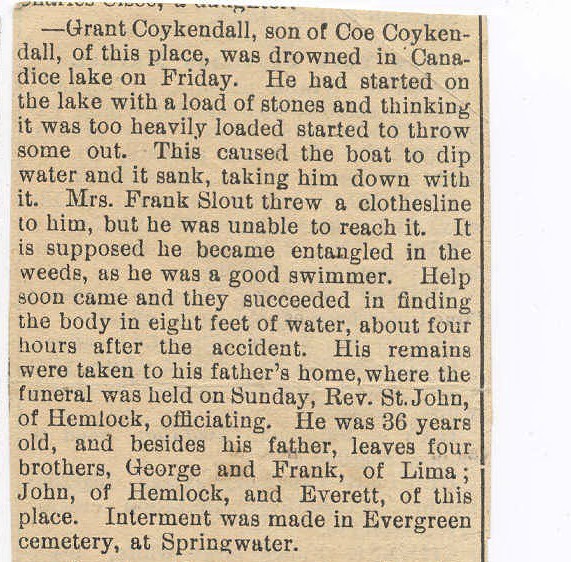The image depicts a close-up of a yellowed, almost brownish, old newspaper clipping with black text. The article solemnly reports the drowning of Grant Kuykendall, aged 36, son of Coe Kuykendall, in Candace Lake on a Friday. The tragic incident occurred while Grant was attempting to lighten an overloaded boat filled with stones by throwing some out, causing the boat to take on water and ultimately sink. Although Mrs. Frank Slout threw a clothesline to him, Grant, a good swimmer, couldn't reach it—it's believed he got entangled in weeds. Help arrived quickly and his body, found in eight feet of water, was recovered about four hours later. His remains were taken to his father’s home, and his funeral was held on Sunday with Reverend St. John of Hemlock officiating. Grant is survived by his father and four brothers: George and Frank of Lima, John of Hemlock, and Everett of their local area. He was laid to rest in Evergreen Cemetery at Springwater.